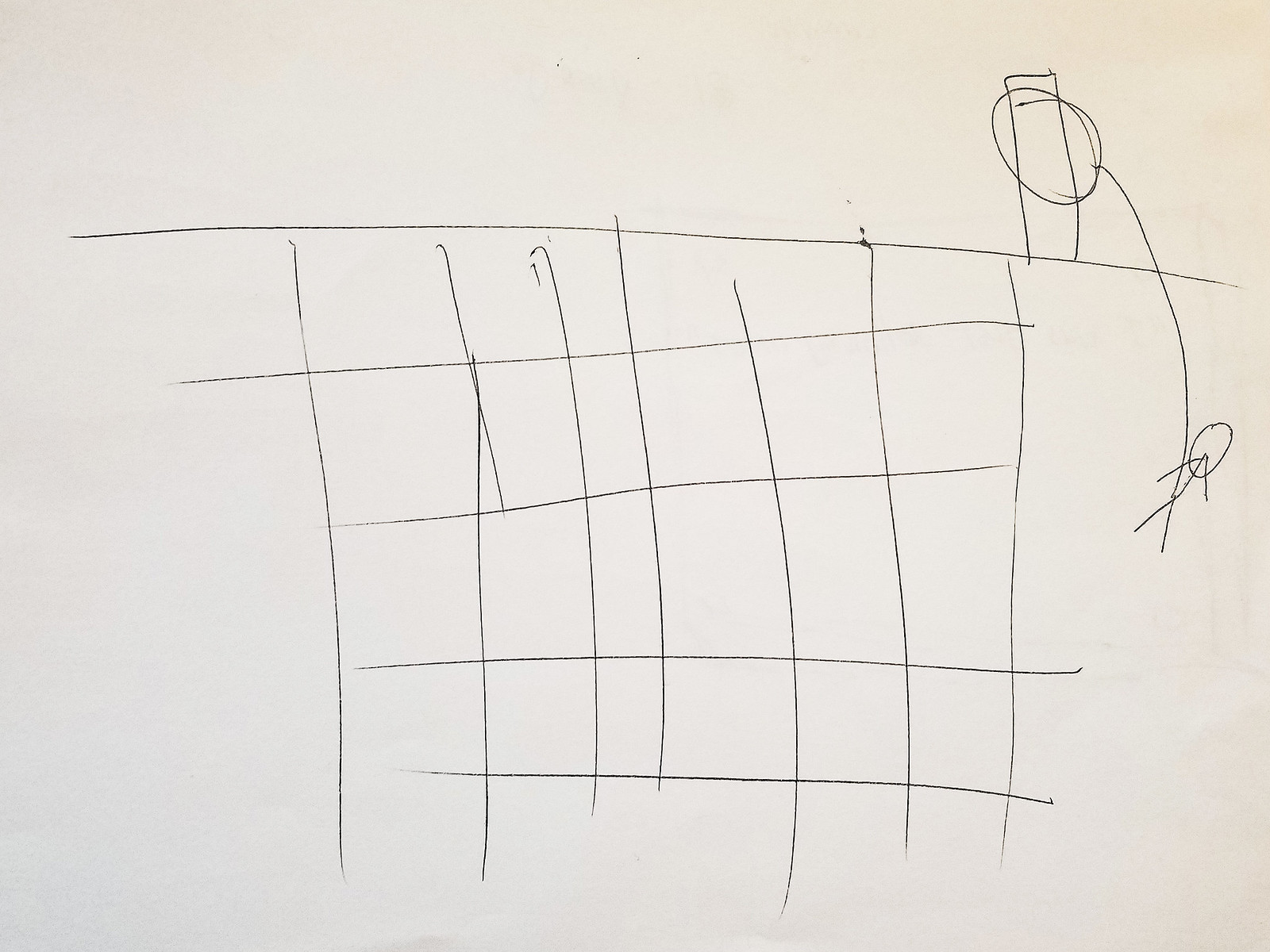This image features a rudimentary line drawing on a somewhat off-white, grainy sheet of paper, displayed in landscape orientation. Dominating the center and extending towards the bottom of the page is a prominent, hand-drawn grid, approximately six columns wide by three to four rows high. This grid stands as the most substantial element in the composition. 

Across the top of the grid, a single horizontal line is discernible. From this line extends a pole-like structure or a rectangular shape towards the upper right section of the page. Encircling this pole is a loosely drawn circle. Suspended from the pole, a vertical line descends, culminating in a simplistic stick figure that appears to be hanging. The stick figure is positioned adjacent to the grid, enhancing the overall crude and minimalistic nature of the drawing.